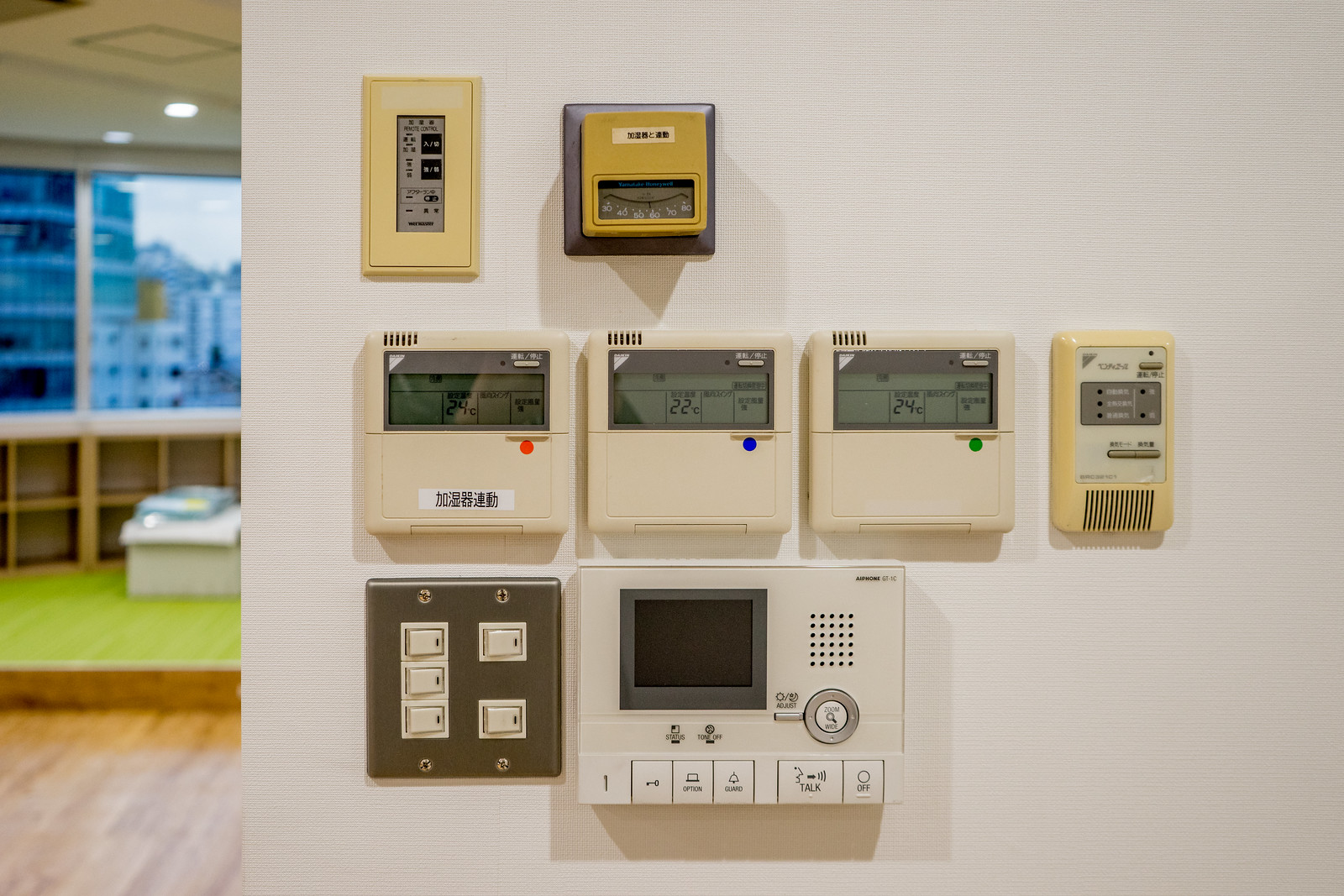This photograph captures a detailed and intriguing wall installation of various meters and thermostats. The white wall is adorned with eight distinct devices, organized in a structured manner. At the top row, there are two units: the left one is a square meter with a mustard yellow cover and a silver rim, while the right one is a vertically oriented rectangular meter featuring a cream-colored case and a gray and black face.

Directly below, there are three identical square meters made from cream-colored plastic, each displaying temperature readings in centigrade on a gray screen. To their right is another rectangular meter, this one pale yellow with a dual-toned gray face.

Beneath this row, a stainless steel plaque is affixed to the wall, showcasing five white flip switches. To the right of this plaque is an additional white plastic thermostat, which has a blank black screen.

Illumination from a bright light casts distinct shadows of these meters onto the wall, adding depth to the scene. In the background, an adjacent room is visible, distinguished by a hardwood floor. One step leads to an area carpeted in lime green, which features built-in bookshelves beneath large picture windows. These windows offer a view of another tall building standing across the way.